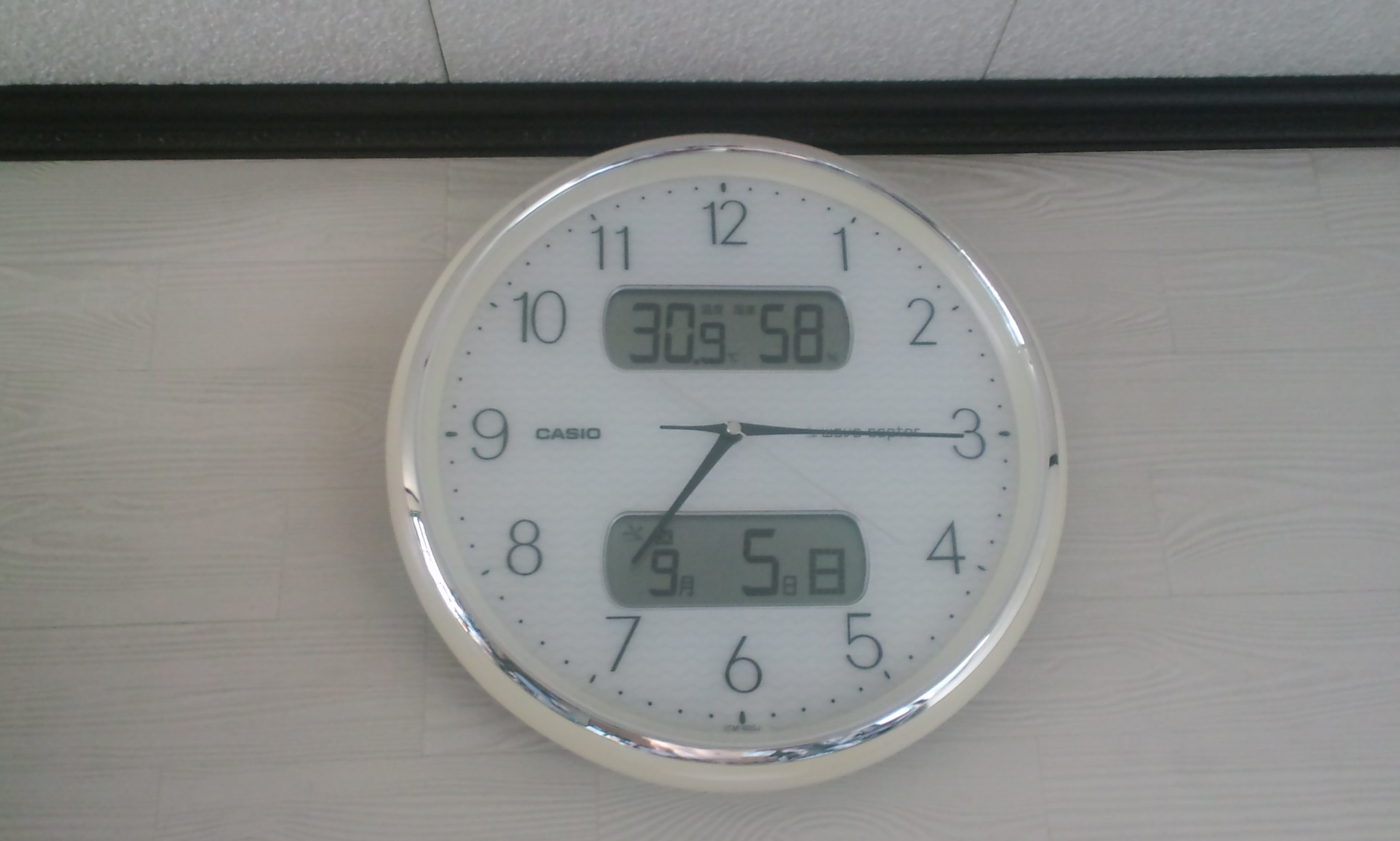This image captures a meticulously detailed round clock that dominates the frame. The clock features a sleek silver circular rim and a protective glass cover. Its face is white, adorned with bold black numbers indicating the hours, and is equipped with thin black hands displaying quarter past seven. Below the numeral twelve, there is a digital inset displaying "30.9 58," while another digital inset located just above the numeral six shows a small "9" followed by a larger "5" and smaller "8." The backdrop consists of a white paneled wall topped with a black trim, which transitions into a white drop ceiling, creating a monochromatic contrast. Overall, the image exudes a minimalist aesthetic with a focus on the clock's intricate design and the surrounding structural elements.